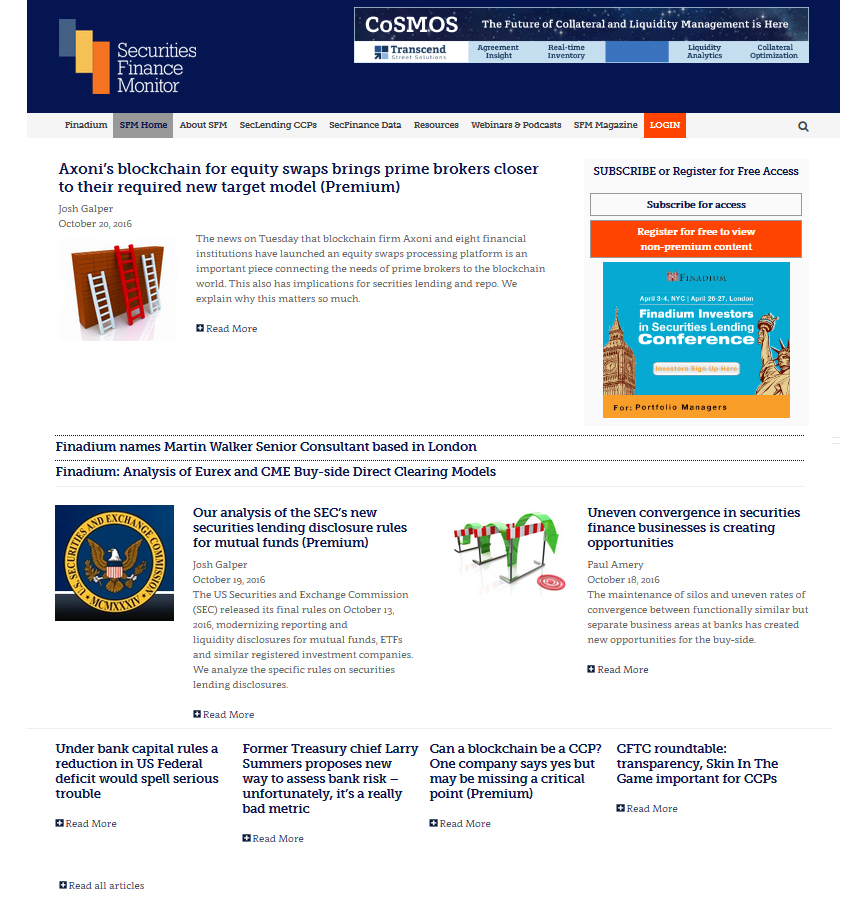**Detailed Caption:**

In the top left corner of the image, there are blue, yellow, and orange bars, symbolizing the interconnected sectors of securities, finance, and monetary systems. Overlaying the cosmic background, these bars represent the future of collateral and liquidity management, emphasizing real-time inventory, liquidity analysis, and collateral optimization. Featured text includes key terms like "consent," "agreement and sign," and promotional sections such as "SPM Home," "About SPM," "SEC Lending," "CCP," "SEC Finance Data," "Resources," "Webinars and Podcasts," and "SFM Magazine."

In the lower portion, the image highlights a significant event dated October 20, 2016, where Josh Galperin discusses the pivotal news from Tuesday about blockchain technologies implemented by Exxon and Afin. The text details the launch of an equity swap processing platform, bridging the gap between private brokers and the blockchain world, ultimately affecting Securities Lending and Real Estate markets.

Additionally, the image mentions Texas advocating for the use of blockchain in equity swaps and introduces notable terms like "Vanadium," "Investors and Creators Lending Conference," and key individuals such as Myron Walker, a tenured consultant based in London, and associations with "Elsevier" and "CME." It also promotes the benefits of subscribing and registering for free to access premium content, elucidating the content's role in shaping modern financial frameworks.

Lastly, the image notes the "Bitesize Direct Credit Model," showcasing a comprehensive view of emerging financial technologies and industry trends.